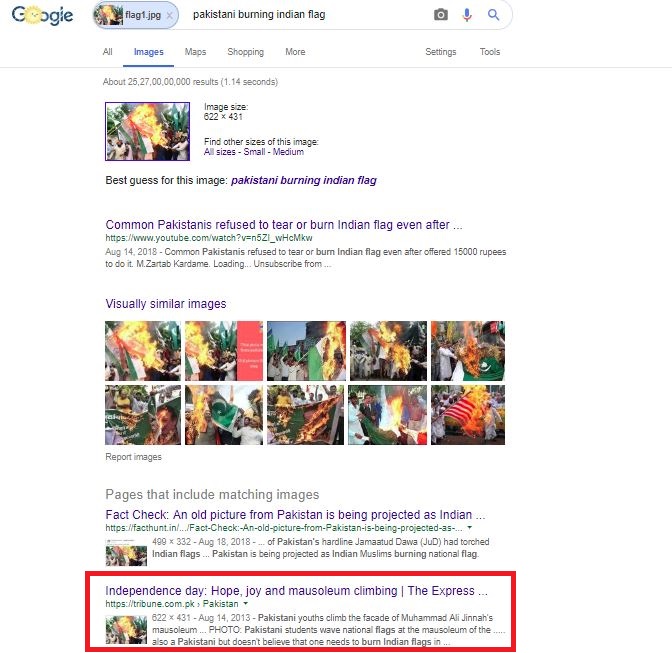**Detailed Caption:**

The image depicts a screenshot of a desktop displaying Google's homepage, featuring a special doodle resembling a clock face. In the search bar, the query "Pakistani burning Indian flag" is entered. Below the search bar, a small thumbnail shows an image named "flag1.jpg," indicating it has been uploaded for a reverse image search, with an option to upload another image using the camera icon.

At the top of the page, the "Images" tab is highlighted among other options like Maps, News, and more settings. The results show approximately 25.27 billion results retrieved in 1.14 seconds. The highlighted image's dimensions read 622 by 431 pixels, with options to find other sizes such as small and medium.

Several search results are listed, the first being a link to a YouTube video. The title "Common Pakistanis Refuse to Tear or Burn Indian Flag Even After 15,000 Rupees Offer" is followed by a URL (https://www.youtube.com/watch?v=n5z1_whcmkw) and a date of August 14, 2018, attributing the report to "Zartab Kardameh." The page indicates the video is loading and offers options to unsubscribe.

Other results include visually similar images of flags burning, with links to report images and pages containing matching images. One notable result is a fact-check article: "An Old Picture from Pakistan is Being Projected as Indian," with its URL truncated (https://facthunt.in/.../fact-check-an-old-picture-from-pakistan-is-being-projected-as...), dated August 18, 2018, and showing an image size of 499 by 332 pixels.

Another result highlights a news piece from the Tribune (https://tribune.com.pk), also dated August 14, 2013, describing Pakistanis climbing the facade of Muhammad Ali Jinnah's mausoleum with national flags. The final result prominently highlighted in red appears most relevant to the search query, hinting at the importance of the historical and current context of flag-burning incidents and public sentiment.